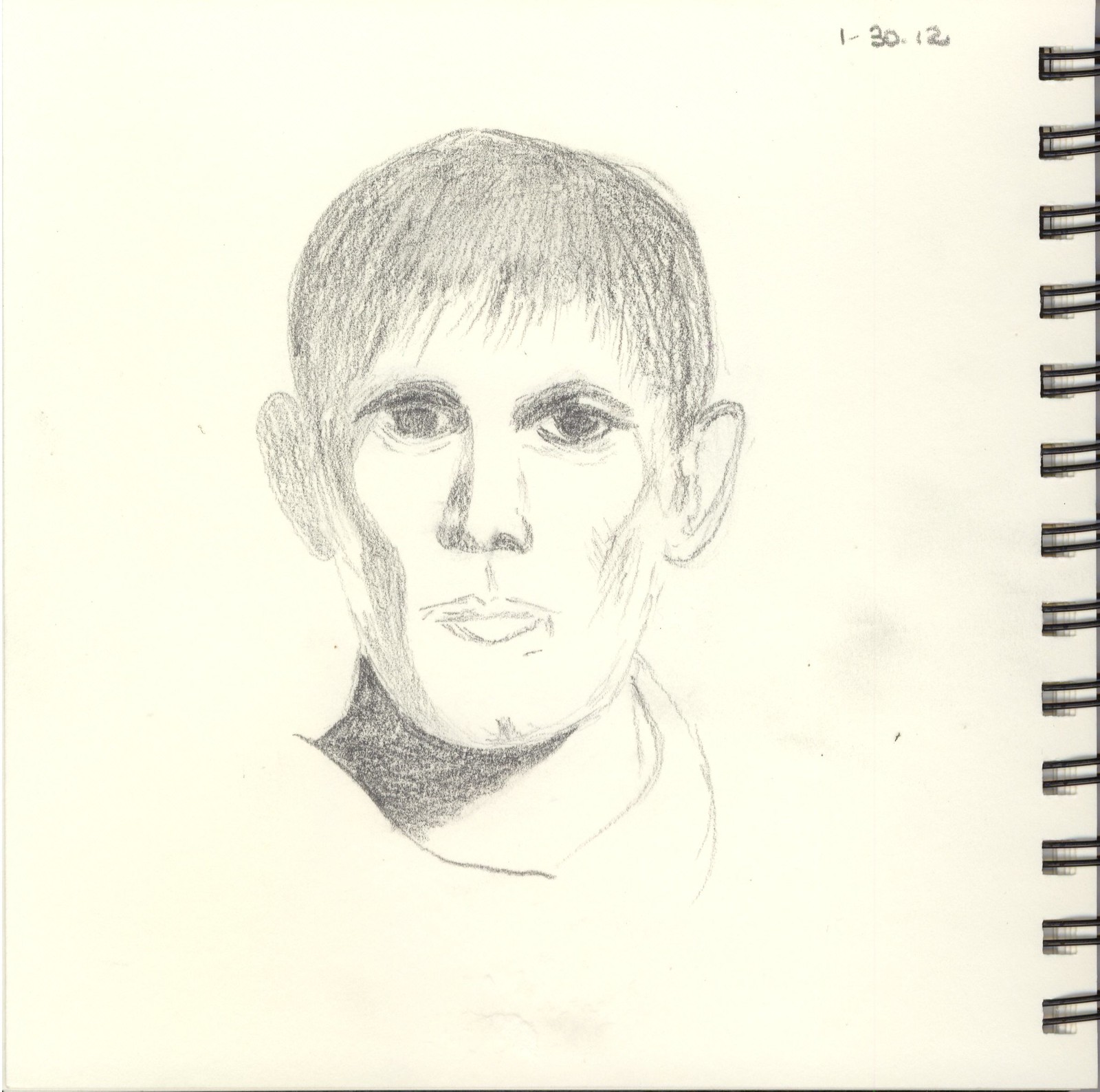This image captures a vertical, rectangular pencil sketch of a man's face on cream-colored sketch paper, bound by a black wire binder on the right-hand side. The drawing, set within a sketchbook, showcases a realistic portrayal of the man, who has short, dark hair with bangs partially covering his forehead. His dark eyes, detailed eyebrows, and pronounced, closed lips are meticulously rendered, accentuating the lifelike quality of the art. There is detailed shading under his chin, brows, and on one side of his face and neck, adding depth to the sketch. His ears are visible, with the right ear appearing darker due to added shading. In the top right corner of the page, the date "1-30-12" is inscribed in pencil. Some slight pencil smudging is noticeable on the white areas of the page. Additionally, an outline of a shirt is subtly suggested, further grounding the drawing in realism.